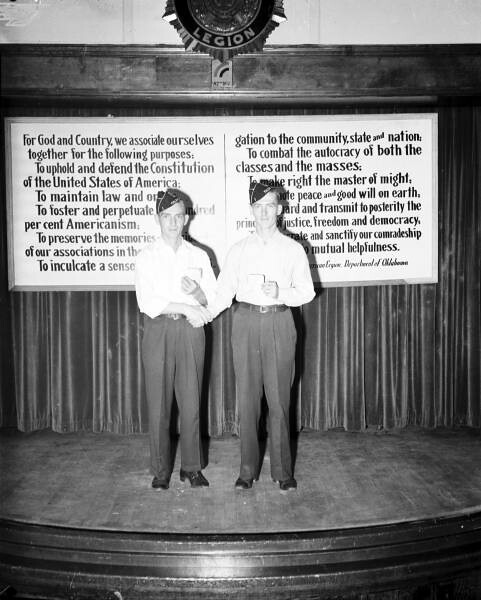In this black and white photograph, two men, who appear to be veterans, are standing on a stage in front of a dark-colored curtain. They are dressed identically in white button-down shirts, tucked into black trousers with belts, and wearing matching side sailor or military-style hats. Both men are holding small white squares in front of them while shaking hands with their other hand, highlighting their camaraderie. Above them, a sign reads, “For God and country, we associate ourselves together…” and is partially obscured by the men's heads. It incorporates a legion emblem, implying this could be related to the American Legion, and speaks to religious and patriotic themes, such as upholding and defending the Constitution of the United States, maintaining law, fostering Americanism, and preserving memories of their associations. Their poised demeanor and identical attire suggest a formal or ceremonial occasion, possibly linked to their service and commitment to community and country.